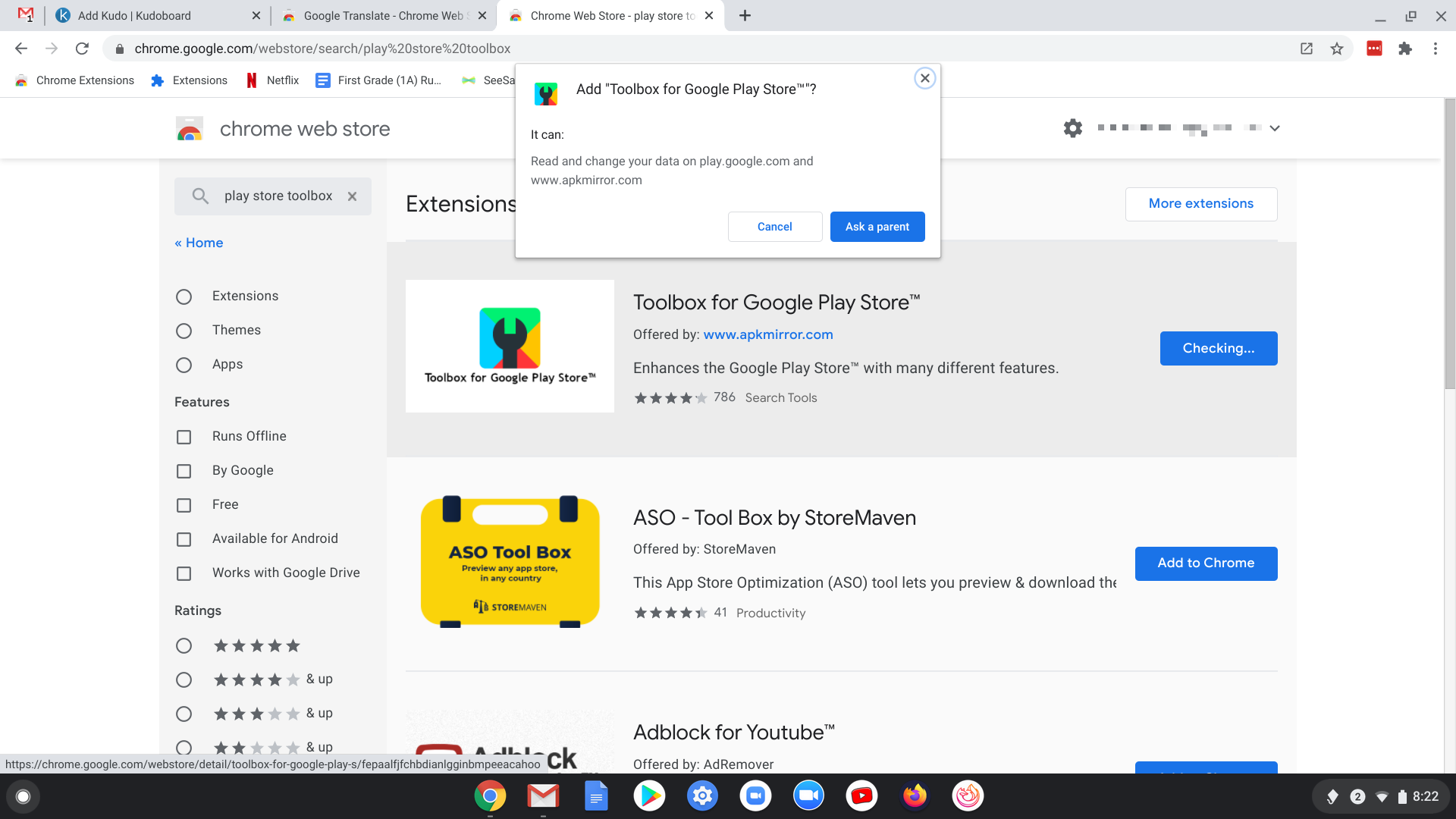The image is a detailed screenshot from a desktop that appears to be a Chromebook, given its distinct interface which is notably different from Windows. The taskbar at the bottom of the screen is black and features a circular white button on the far left, indicating the app launcher. Centered along the taskbar are the pinned applications, which include icons for Google Chrome, Gmail, Google Docs, the Google Play Store, Settings, FaceTime (or a similar video call app), YouTube, Firefox, and another unidentified app, predominantly showcasing Google's suite of tools.

Within the screenshot, Google Chrome is active, displaying the Google Chrome Web Store. The user is in the process of adding an extension called "Toolbox for Google Play Store." They have already searched for this tool and are on the results page. The primary focus is on the blue "Add to Chrome" button that has been clicked, changing its state to "Checking...".

An overlaid white pop-up appears, prompting the user to add the "Toolbox for Google Play Store" extension, detailing that this extension can read and modify data on PlayGoogle.com and www.apkmirror.com. Two options are available at the bottom of the pop-up: "Cancel" or "Ask a parent," with the latter highlighted in a blue button. The entire page has a clean, white background, adhering to Google's standard light mode theme.